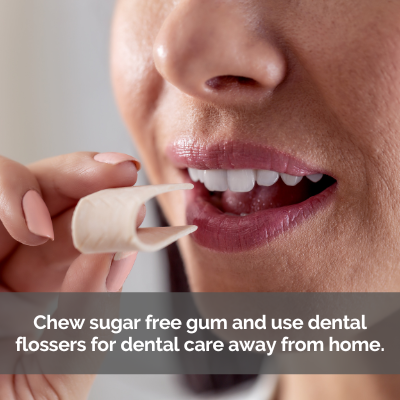This photograph presents a close-up view of a woman's face, focusing on the area from her nose down to her chin. She wears a hint of red lipstick and displays exceptionally white teeth. Her mouth is slightly open, suggesting she is about to chew a piece of gum. Her right hand, adorned with light pink nail polish, gently folds the piece of gum into a U-shape, poised to insert it into her mouth. The background of the image is plain and somewhat blurry, drawing attention to the act of chewing gum. At the bottom of the photograph, a semi-transparent gray banner with white text offers dental advice: "Chew sugar-free gum and use dental flossers for dental care away from home."